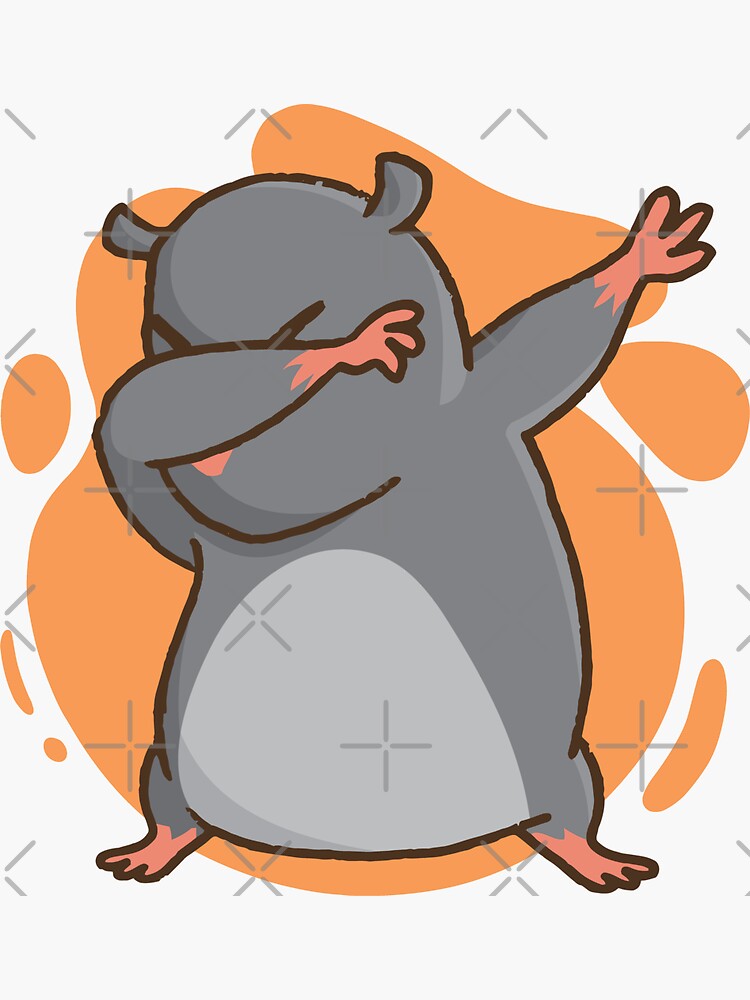The image is a child-like, animated rodent depicted in a vector, cartoon style. This character, which resembles a mouse, gerbil, or hamster, is primarily dark grey with a light grey stomach. Detailed features include pink hands, feet, and nose, with black outlines accentuating its form. The rodent is striking a dabbing pose, with one arm bent over its face and the other extended outward, while its legs are slightly apart. The background displays an abstract, splotchy orange design against a white backdrop, overlaid with a grey cross pattern likely meant to serve as a digital watermark to prevent unauthorized use. The overall scene is cute and lively, capturing the playful motion of the rodent.